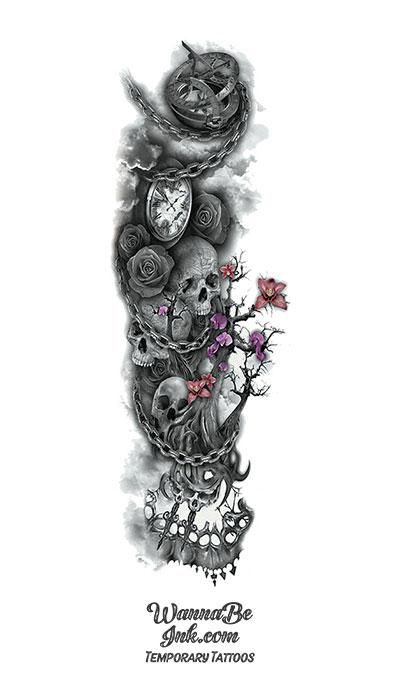The image is an elaborate drawing likely intended as a template for a temporary tattoo, showcased without a defined border against a white background. This long, vertical design starts at the top with an old-fashioned compass or sundial attached to a chain. Progressing downward, the illustration features a jack-o-lantern, various skulls intertwined with black roses and thorny trees, creating an intricate pattern. The composition includes both colored and monochrome elements, such as the black and white skulls, pocket watches, and roses, juxtaposed with vibrant pink and purple flowers. Chains wrap around the skulls and pocket watches, adding a steampunk flair to the design. At the base of this stacked image, the text "wannabeink.com temporary tattoos" is prominently displayed, indicating that this detailed and ornate artwork is an advertisement for a temporary tattoo company.